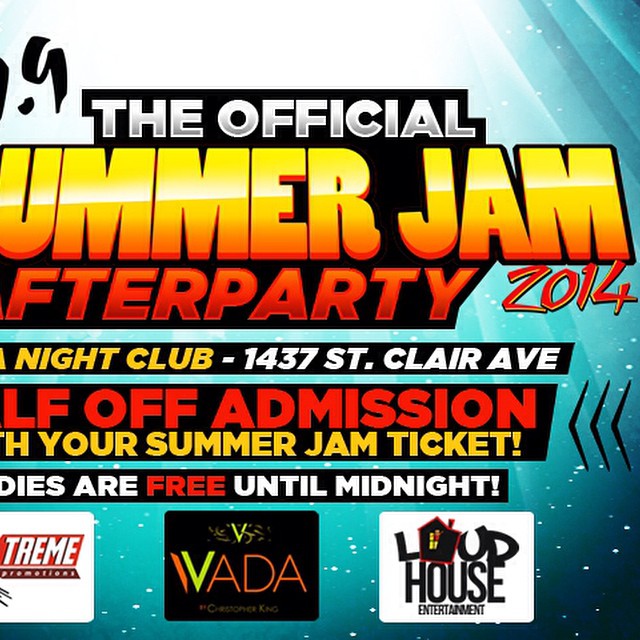This vibrant and colorful advertisement, likely designed for the internet or a magazine, features a partially cropped image promoting the "Official Summer Jam After Party 2014" at Night Club 1437 St. Clair Avenue. The ad has a blue background that fades to bright white at the top, resembling an ocean with highlights, adding a lively and festive touch. The prominent, bold, and 3D-like title is written in vibrant yellow, red, and orange lettering. It mentions that admission is half off with your Summer Jam ticket and that entry is free until midnight, although some of the details are cut off. The bottom section of the ad showcases three sponsor logos: one partially visible with the letters "TREME", another with a black background displaying "VADA" in bright green and orange, and the third, "Loud House Entertainment", with a white background and a house icon replacing the 'O' in 'Loud'. The ad also features little white specks throughout, enhancing the vibrant layout.